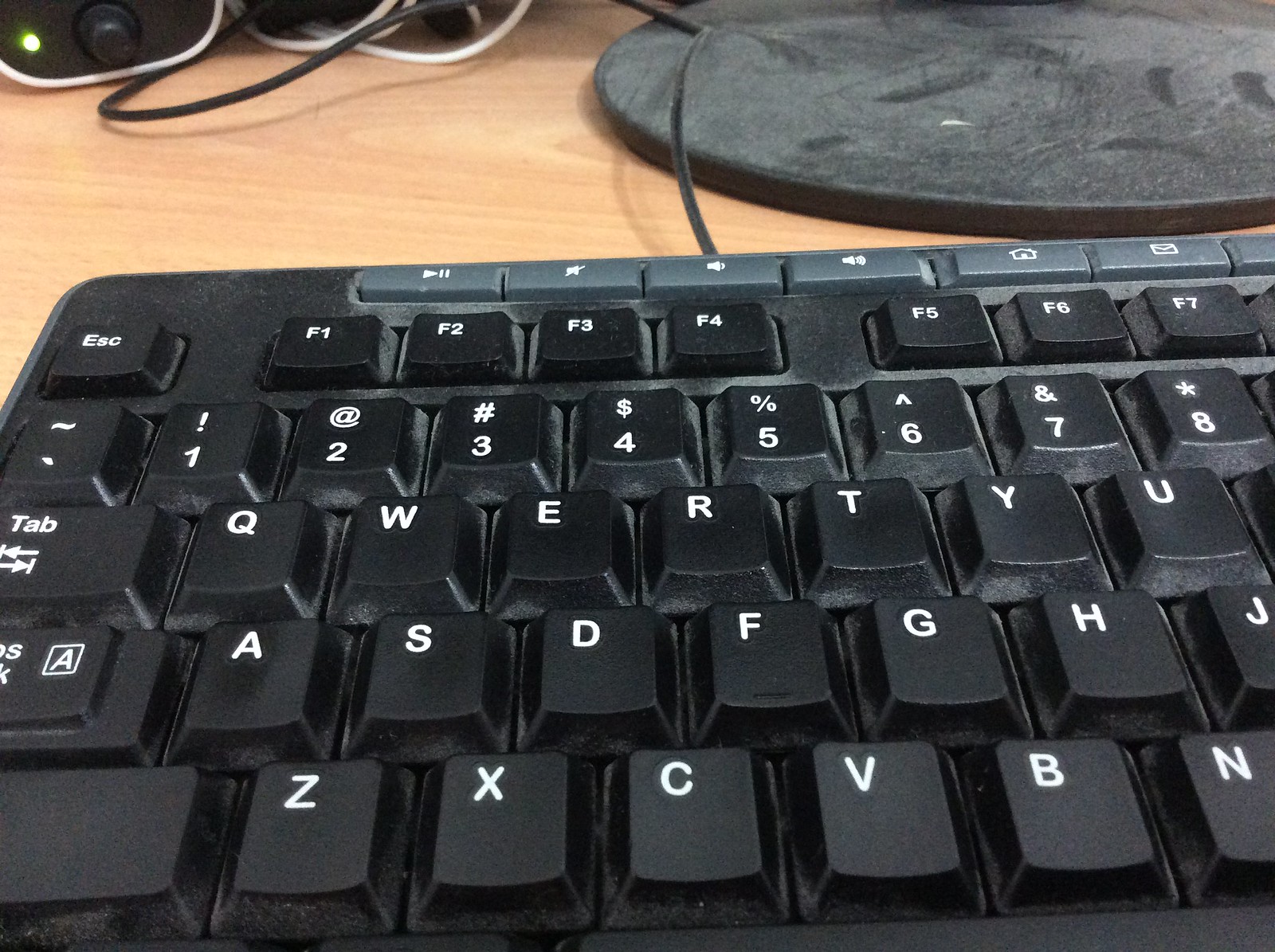The photograph showcases the upper left portion of a black QWERTY computer keyboard with white lettering, situated on a light-colored wooden desk. The visible keyboard section includes the keys from Q up to U on the top row, A to J in the middle row, Z to N in the bottom row, and extends to the number 8 and the F7 key. At the very top, there are gray buttons with additional functions such as play/pause, mute, volume controls, home, and an envelope icon for email. To the upper right, there's a very dusty circular plastic base likely for a monitor. In the upper left, there's a rounded rectangle-shaped device resembling a speaker with a black faceplate, white outline, black knob, and a green light illuminated. The desk also has visible black and white wires scattered around the area, adding to the cluttered setup.